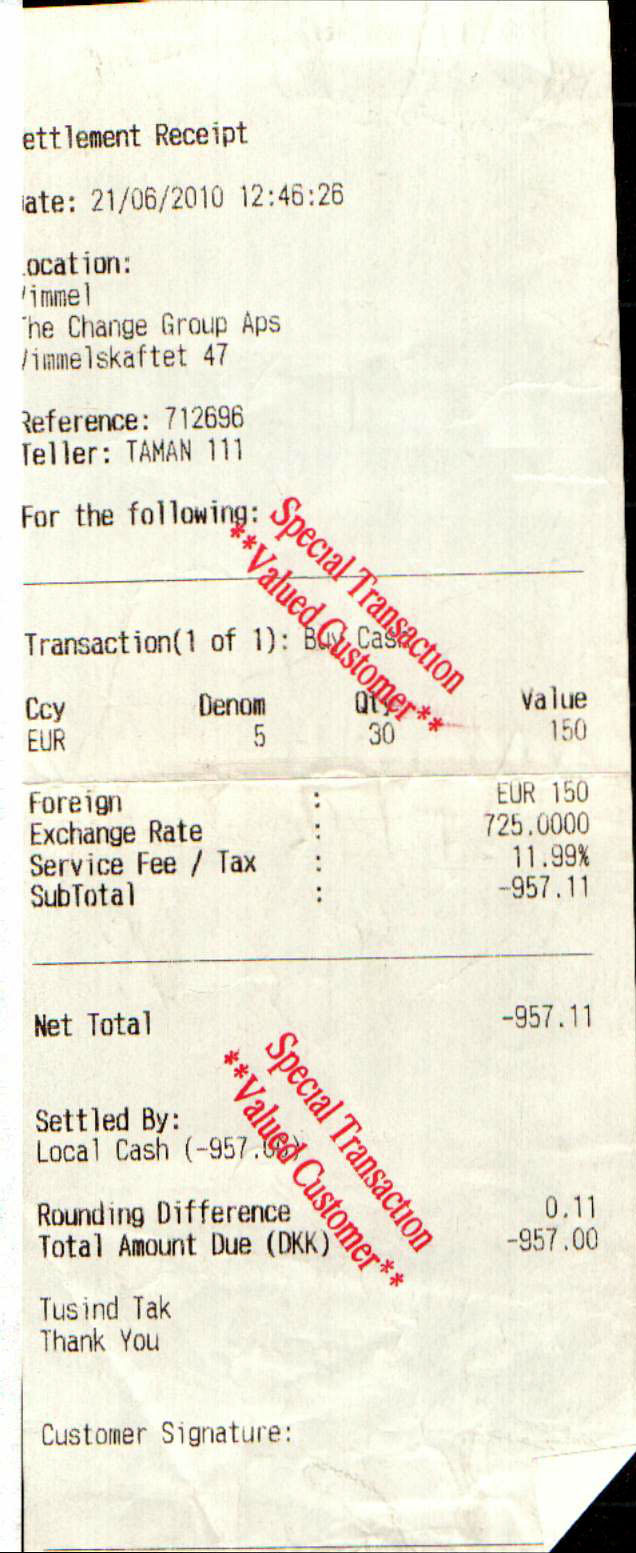The image depicts an aged and wrinkled receipt that has been flattened out. The receipt is titled "Settlement Receipt" in black text at the top, though the paper shows signs of wear, appearing off-white and faded. The transaction details date back to 21-06-2010 at 12:46:26. Key information includes the location identified as part of "The Change Group" apps and a reference number, 712696, with teller Taman111 facilitating the transaction, indicated as "1 of 1".

The receipt itemizes the transaction involving euros:
- Currency: Euro
- Denomination: 5
- Quantity: 30
- Value: 150
- Foreign currency value: 150 Euros
- Exchange rate: 7.25
- Service fee and tax: 11.99%
- Subtotal: -957.11
- Net total: -957.11
- Settled by local cash with a rounding difference of 0.11, resulting in a total amount due of -957.11

Additionally, there are red stamps on the receipt stating "Special Transaction, Valued Customer" prominently stamped twice—once in the middle and again towards the bottom of the document. Further details such as a "customer signature" space are noted at the bottom of the receipt.